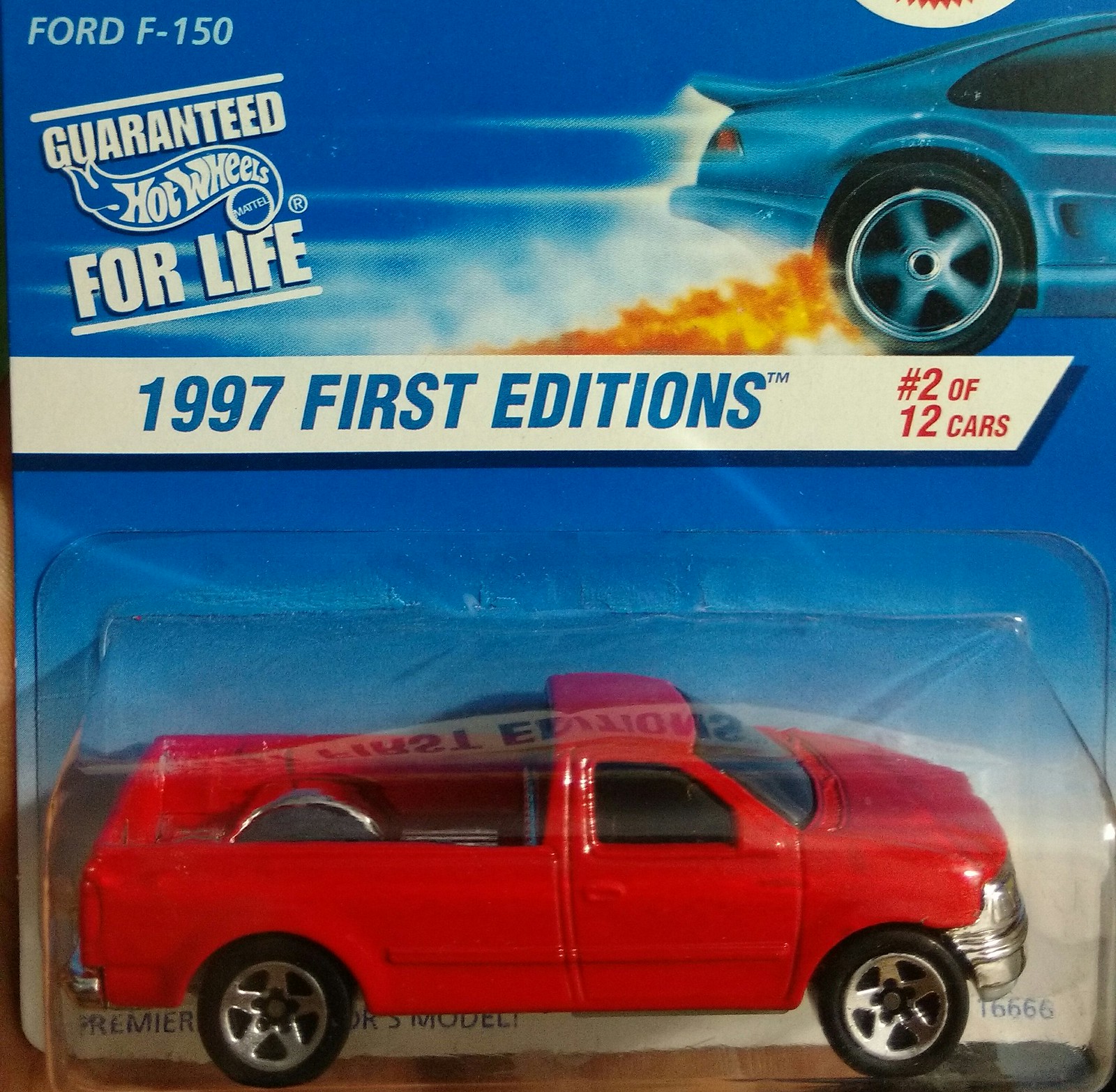The image features a 1997 first edition Hot Wheels toy car, specifically a red Ford F-150 pickup truck, marked as number 2 out of 12 cars. The toy is encased in a plastic cover, which is attached to packaging made of a blue piece of cardboard that transitions to white towards the bottom. The packaging prominently displays a blue race car with fiery effects around its wheels. Also visible on the packaging is a "Guaranteed Hot Wheels for Life" logo by Mattel. The product is photographed on a wooden desk. The truck itself has black wheels and silver details on the front and bed.